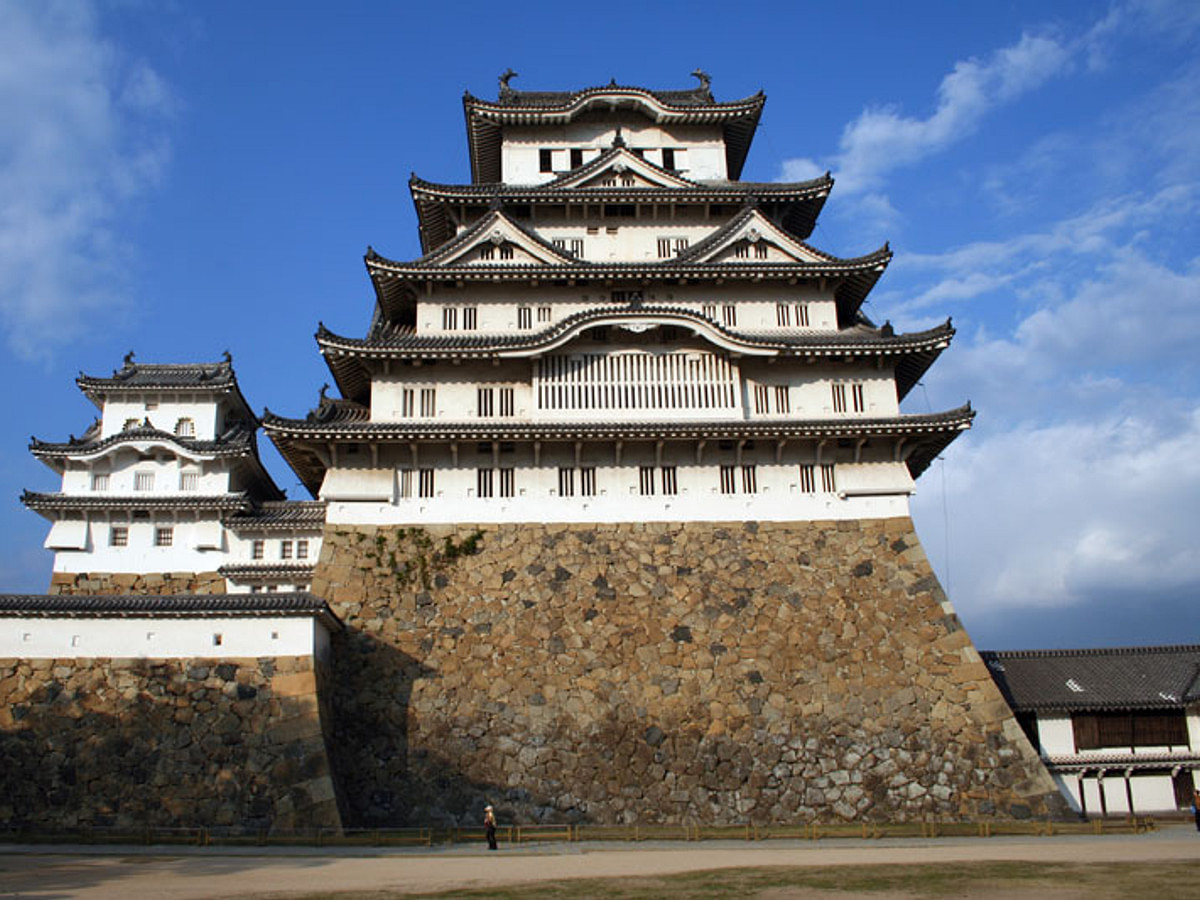In this daytime photograph set against a bright blue sky with wispy clouds, we see a striking depiction of traditional Japanese architecture. The focal point is a substantial pagoda-style building, distinguished by its white walls and stacked black rooftops that taper as they ascend, showcasing characteristic curved roofline features and multiple peaks. The building is comprised of five to six layers, each smaller than the one below, creating a visually compelling tiered effect. It stands majestically atop a fortified stone foundation, reminiscent of a pyramid, which rises approximately 50 to 60 feet high, composed of grey and brown rocks. There is no walking area or platform around the base, giving it an imposing and isolated presence.

To the left of the main structure, there is a smaller three-layered building of similar architectural style. Extending on the right, closer to ground level, stands a two-story building with flat rooftops. A road runs across the foreground beneath the tall stone wall of the large building, and a small person is visible, emphasizing the grand scale and height of the structure. This scene suggests the presence of an ancient fortress or possibly a historic residential complex, surrounded by other buildings that echo its distinct Asian flair.